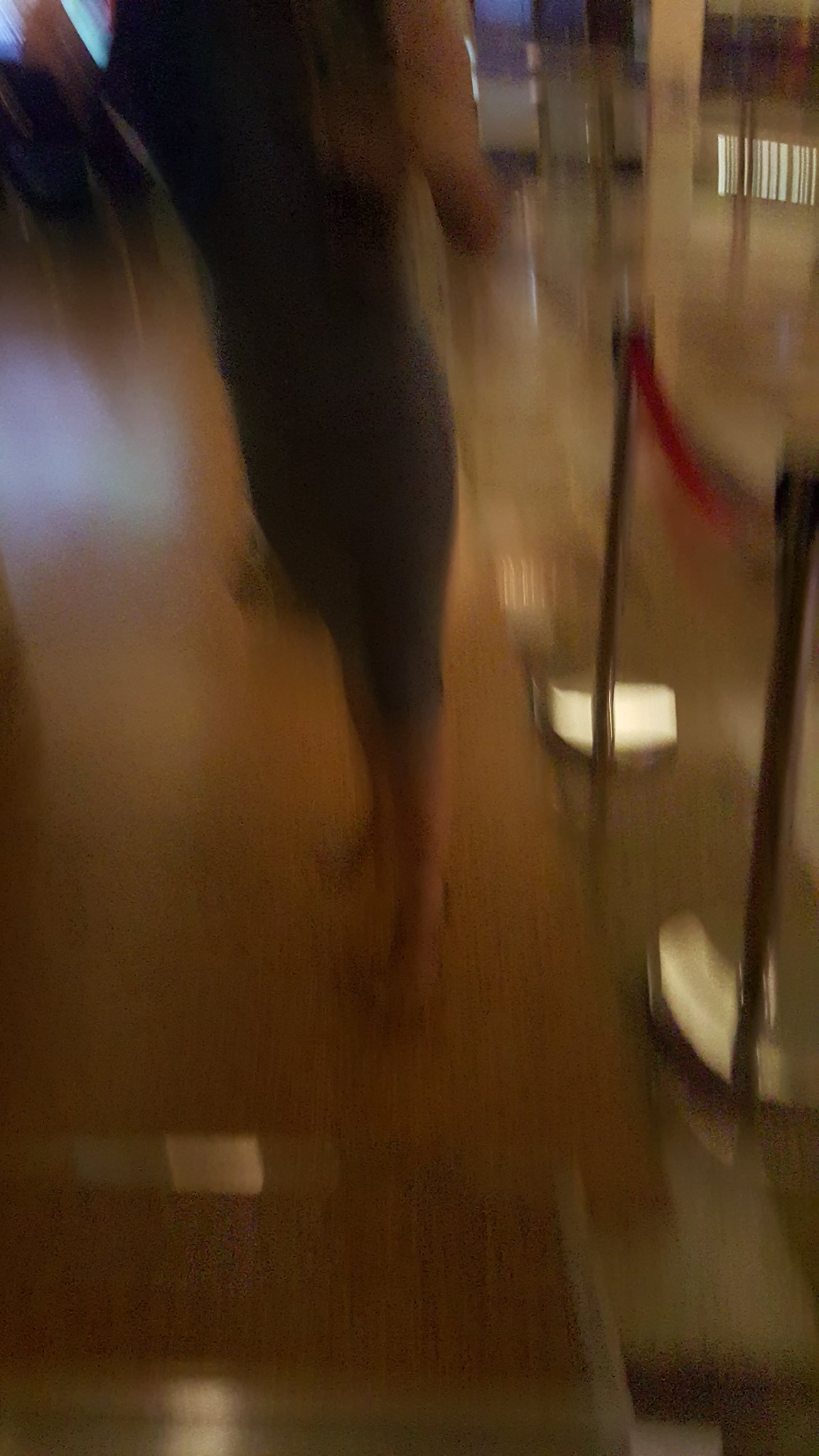This photograph, though blurry, captures a scene with a central figure, a woman who appears to be Caucasian. She stands facing left, attired in form-fitting black clothing with cropped pants that reveal her high heels. Her ensemble is sleeveless, exposing her bare arm. To her right, we notice a couple of silver cylindrical poles protruding from the ground. The background in the upper right showcases a window, hinting at an interior setting, and the woman is positioned on a brown wooden floor. Additionally, in the upper left corner, there is another indistinct figure walking towards her, accompanied by light reflections both in front of them and in the lower left corner of the image.